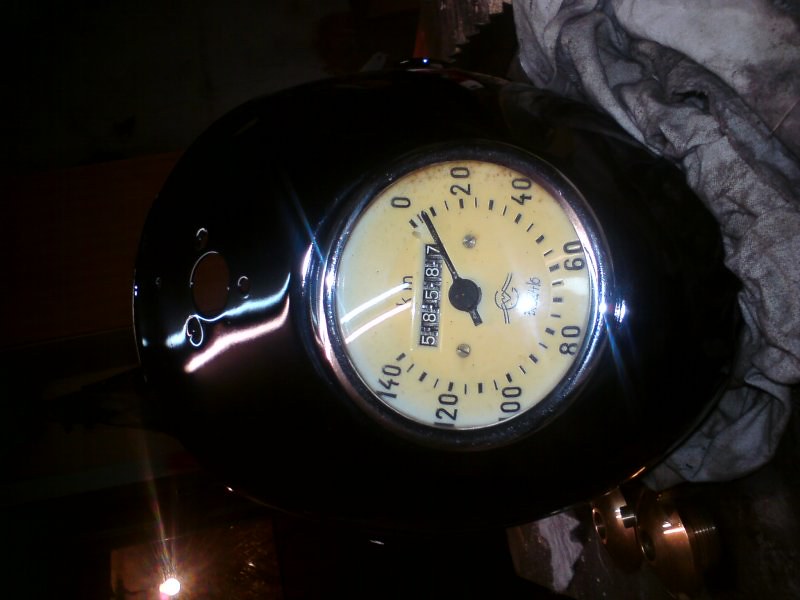The image features a multi-tonal, abstract background that transitions from gray in the upper left corner to brown, followed by darker shades of gray with hints of green and greenish-brown towards the bottom. Central to the composition, a light fixture with a black outer casing encases a bulb outlined in a silver circle. The interior of the bulb glows yellow, subtly tinged with blue-green around the edges. This illumination highlights a dial with numbers and a single hand that moves between them. Surrounding the numbers are a combination of thick and thin dashes. Below this setup, a black counter displays the number "588587" in white text. On the right side of the image, there's a fabric with a white, light gray, and black pattern. Underneath this fabric, the background transitions to black with a coppery hue slightly to the left.